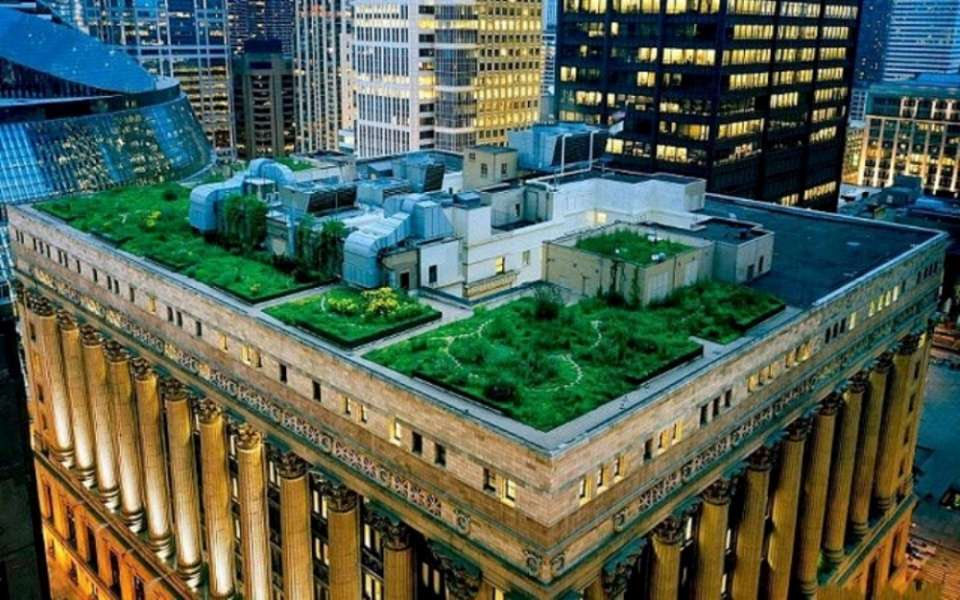This image showcases a rooftop garden on a vintage-style tall building, likely situated in a bustling cityscape reminiscent of New York. The main focus is on the rooftop, where plots of grass and planter boxes with blooming yellow flowers add a touch of green to the urban setting. The rooftop garden is sectioned off by walkways, forming square or diamond-shaped patterns depending on the angle. Various mechanical structures and doorways leading to staircases can also be seen, hinting at the building's older architecture with its columns and stone facades.

As dusk settles in, the city comes alive with the twinkle of lights from numerous office buildings and apartments in the background. Skyscrapers stretch high into the twilight blue sky, their myriad windows casting a warm glow. The foreground rooftop appears slightly neglected, with overgrown patches of grass set against areas covered with tar. The garden’s vibrancy contrasts the otherwise industrial appearance, creating a serene escape amidst the urban sprawl. A crosswalk is faintly visible in the lower right corner, adding another layer of depth to this compelling cityscape.